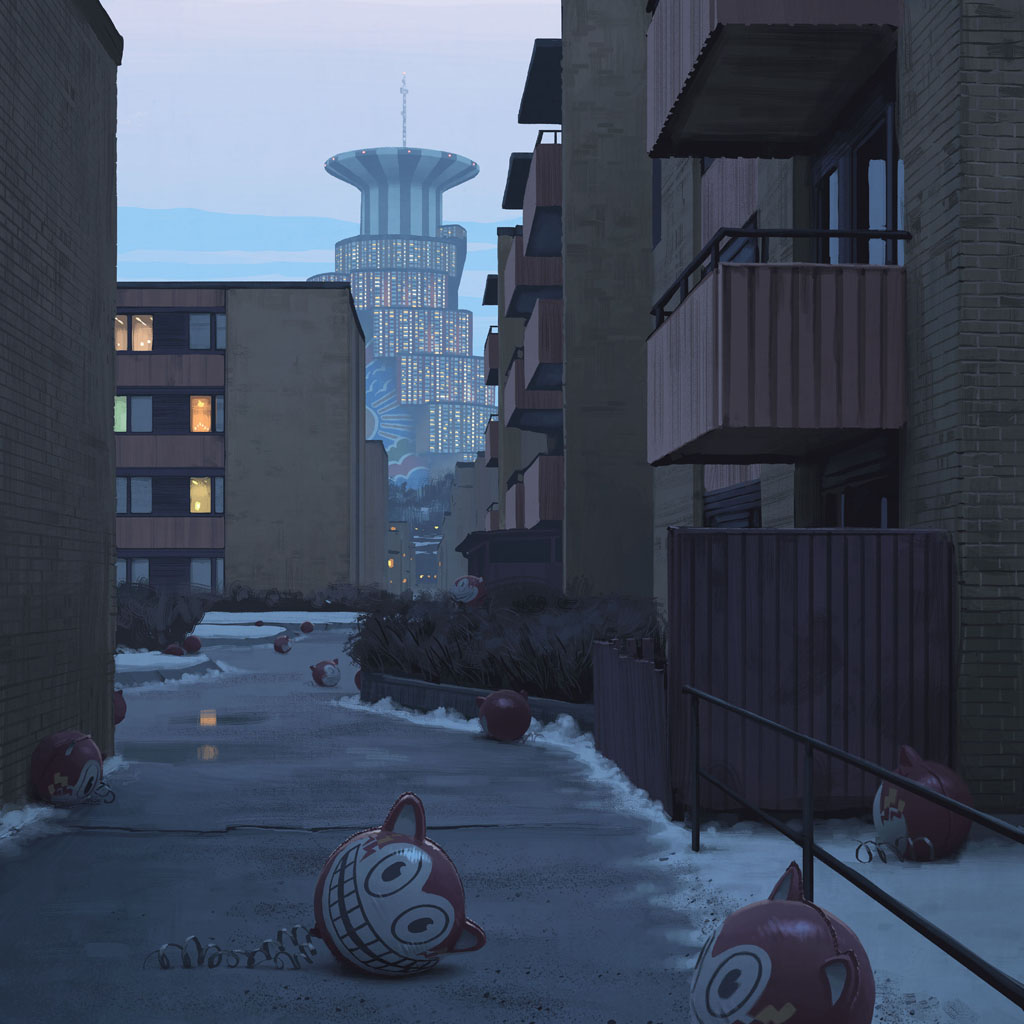The image likely depicts a cityscape, possibly in Japan, viewed from one end of a snow-lined sidewalk amidst an apartment complex. The sidewalk is littered with large, red, grinning cat heads with pointy ears, standing on twisted springs, resembling broken playground equipment. These scattered cat head structures, complete with handlebars, seem out of place, giving the scene an eerie yet playful aesthetic. The apartment buildings on either side feature outside patios on each floor, some with lights on, hinting at habitation, yet the area is devoid of people. In the background, a towering, unusually shaped building with staggered levels rises, resembling an inverted top hat. Part of this building is adorned with a mural or decoration displaying a sun with multicolored rays in green, red, and blue. The odd combination of playful, surreal elements and residential architecture creates a vivid and almost dreamlike urban scenery.